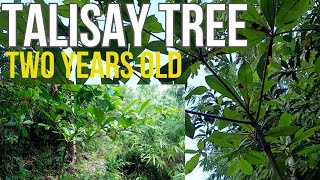The image is a small composite photograph featuring two distinct perspectives of a Talisay tree, both labeled in large block letters that span about a fifth of the image. The text reads "Talisay tree" in prominent white font, with an additional yellow caption underneath stating "two years old." The left side of the image provides a dense close-up view of multiple Talisay trees from ground level, capturing a mix of stems and roots amidst thick undergrowth. On the right side, the photograph offers an upward glance from the ground, showcasing the underside of the tree's canopy with its slender branches and large, green, magnolia-shaped leaves. The sky can be seen through the gaps between the leaves, adding a backdrop to the detailed foliage. Smaller leaves from neighboring trees are also visible in the background, contributing to the tropical ambiance of the composition.